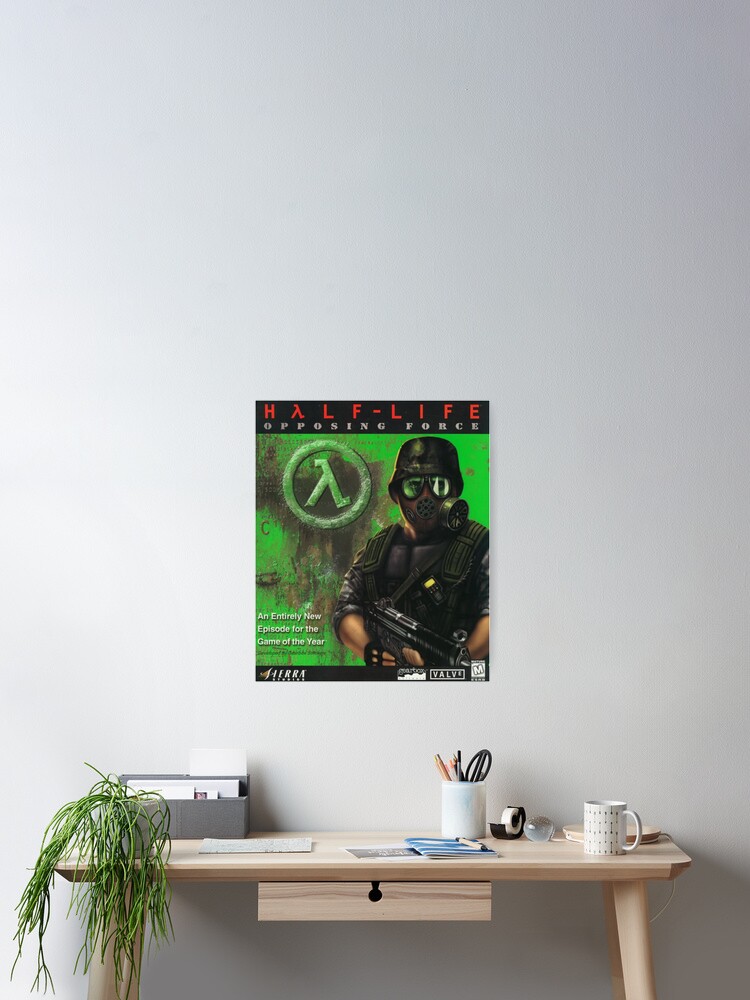The image depicts a well-lit, clear interior space featuring a neatly arranged birch wood office desk. The desk, light brown in color, houses various items such as a desk lamp, a cup of coffee, a small plant, paperwork, and a cup containing pencils and scissors. Centrally placed on the desk is a small pull-out drawer. Mounted on the wall above the desk is a vibrant green game poster for "Half-Life: Opposing Force," showcasing an image of a soldier beside a circular logo with the letter A inside it. The room is brightly illuminated, enhancing the visibility and details of the scene.